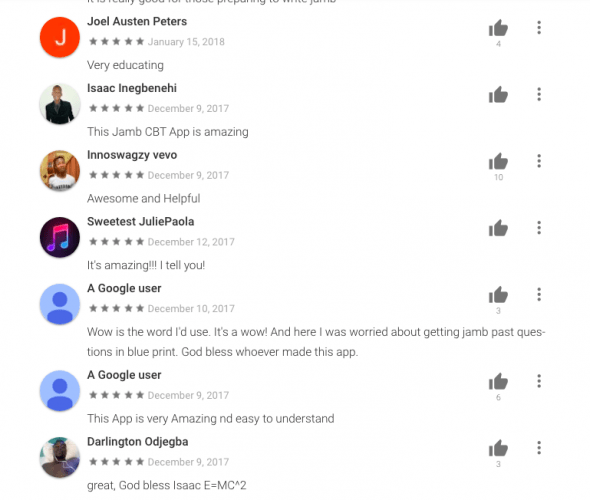Screenshot from a website displaying user reviews for an unidentified application:

- Joel Austin Peters: ★★★★★ (January 15, 2018) - "Very educating."
- Isaac Inigbenehi: ★★★★★ (December 9, 2017) - "This Jam CBT app is amazing."
- EnoSwagZVivo: ★★★★★ (December 9, 2017) - "Awesome and helpful."
- SweetestJuliePaola: ★★★★★ (December 12, 2017) - "It's amazing, I tell you."
- A Google user: ★★★★★ (December 10, 2017) - "Wow is the word I'd use. It's a wow. And here I was worried about getting past JAM questions in Blueprint. God bless whoever made this app."
- A Google user: ★★★★★ (December 9, 2017) - "This app is very amazing and easy to understand."
- Darlington Ojegba: ★★★★★ (December 9, 2017) - "Great, God bless Isaac. E equals MC squared."

To the right, there is a vertical column of thumbs up icons with the following counts from top to bottom: 4, 1, 10, 1, 3, 6, 3.